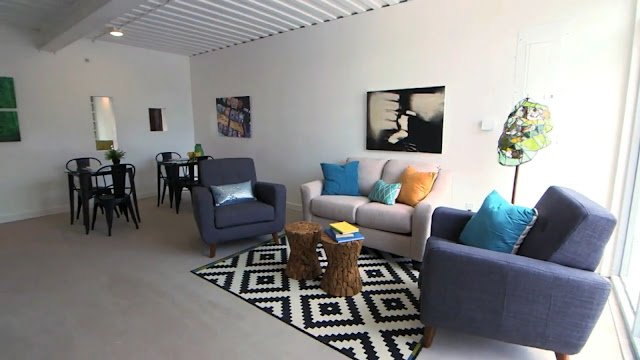The living room features a white ceiling adorned with subtle white straps running horizontally, complemented by a central white beam. The walls on the back and side are painted white, providing a clean and minimalist backdrop. On the right side, there is a large window that may either be a sliding glass door or a stationary window, allowing plenty of natural light to flood the room.

The flooring is a light gray, topped with a black-outlined carpet featuring a white and gray checkered pattern. Two round, brown log-like tables serve as centerpieces, with a blue and yellow book upright on the right one. 

Two dark purple chairs are positioned opposite each other; the chair on the left has a silver cushion, while the one on the right boasts a blue and gray cushion. A beige couch sits centrally, adorned with a variety of pillows: a blue pillow on the right, a green and light bluish pillow in the middle, and an orange pillow on the left.

The room’s decor includes a pair of artworks: two gray and black paintings with shades of white in the middle and another square painting to the left. A chic white light fixture hangs to the right, and there is a distinctive lamp featuring brown, green, and bluish hues with a black bulb base.

Towards the back on the left side, there are two smaller tables accompanied by black chairs, with a mirror positioned behind them. Another square painting is situated to the right. A green element, possibly another window or painting, is located on the left side, adding an additional splash of color to the otherwise neutral palette.